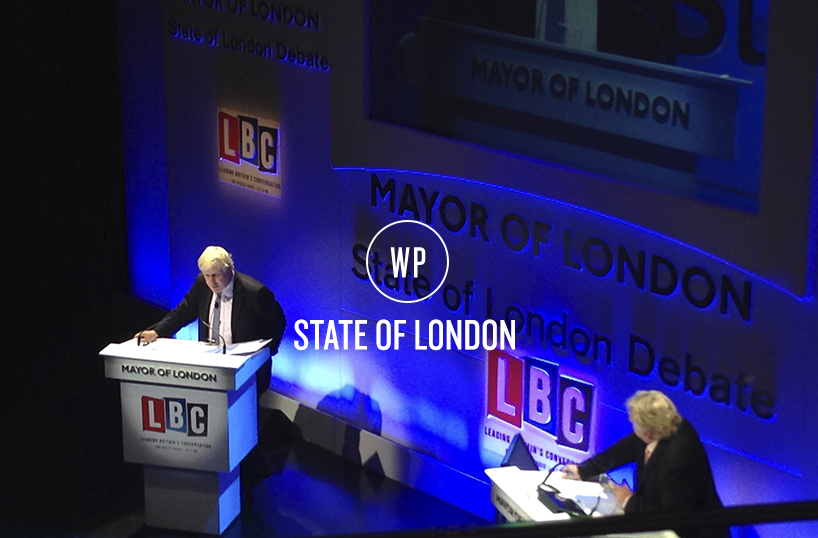The photograph captures a dramatic moment from the Mayor of London, State of London debate, featuring two mayoral candidates on a dimly lit stage. Both candidates, wearing black suits and white shirts, are positioned behind sleek, white podiums adorned with the "LBC" logo, which uses red, blue, and black rectangles for its lettering. The "Mayor of London" and "State of London" inscriptions on the podiums and the backdrop emphasize the political significance of the event. The stage lighting casts a blue hue over the scene, adding to the intensity. The camera angle is slightly askew, providing a clearer view of the candidate on the left, who appears more prominent, while the candidate on the right is seen over the shoulder. An icon in the middle foreground of the image reads "WP" above "State of London," further branding the event as a major debate for London's mayoral election.